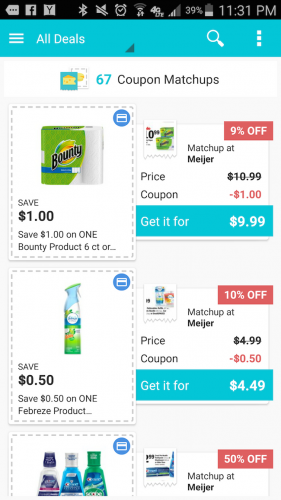In this image, a cellphone screen displays a variety of icons and information. At the top of the screen, there's a status bar showing icons for Facebook, Bluetooth, a price tag, a sound alarm, and signal bars, with a 39% battery charge and the time 11:31 PM. Below the status bar, a turquoise strip labeled "All Deals" transitions to a black strip with white text, followed by a blue strip with white text. This blue strip features three horizontal bars on the left, labeled "All Deals", and includes a magnifying glass icon for search and three vertically aligned dots.

The main content of the screen consists of a list of coupons. The header indicates "67 Coupon Matchups" with the number '67' in turquoise and the words 'Coupon Matchups' in black. Along the left side, there are visible coupon listings, some of which appear to be partially clipped off. The first full coupon on the left promotes "Bounty", advertising a savings of one dollar on a single six-count Bounty product. On the right, another coupon details a price matchup at "Meijer", stating a 9% discount, bringing the final price to $9.99 after applying the coupon, down from the original $10.99.